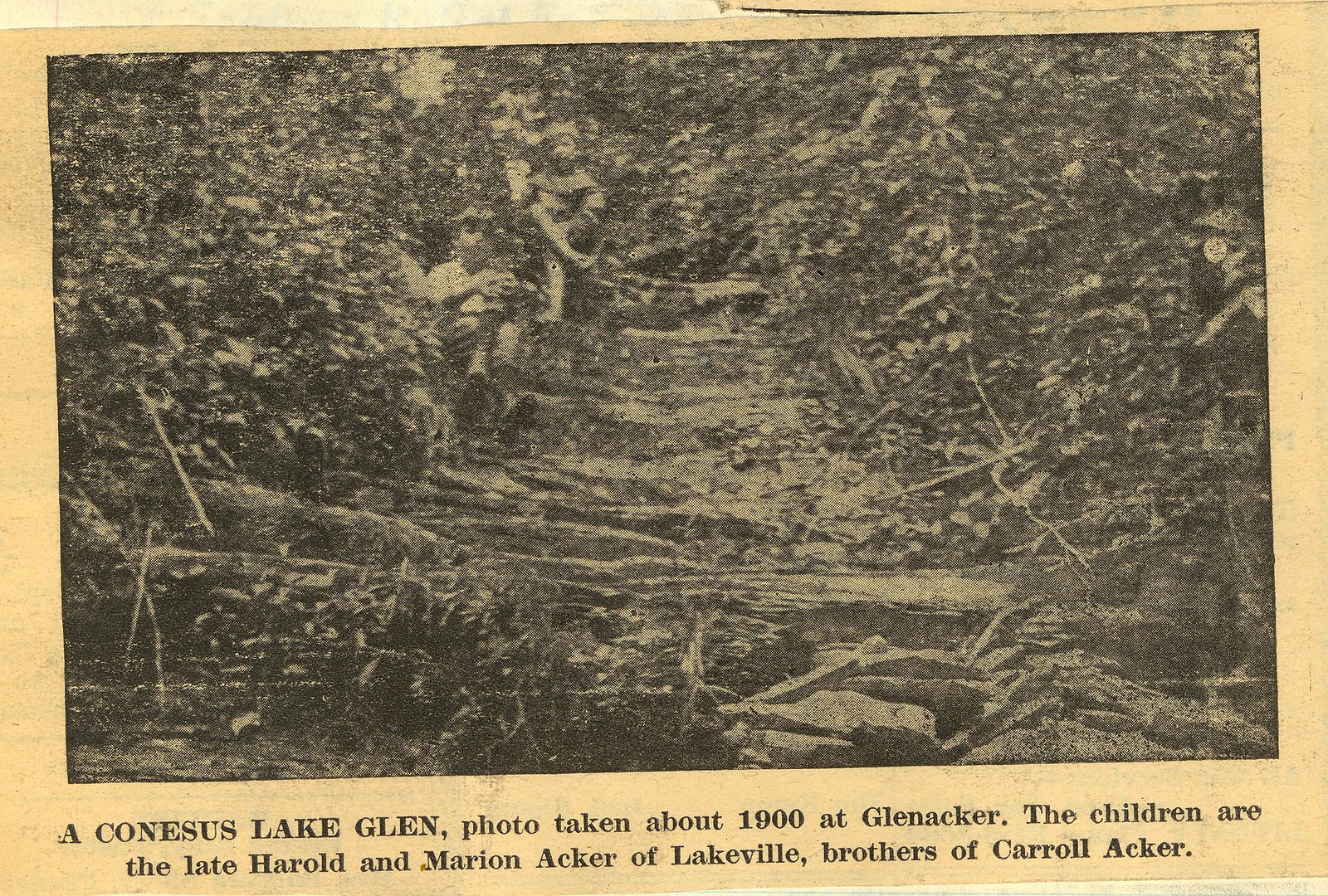The image appears to be an aged, black-and-white photograph, possibly clipped from a very old newspaper, set against a tannish background with a light brown border. The overall quality is poor and blurred, making the scene difficult to discern clearly. The central focus reveals two children seated outdoors on stumps or on the ground, surrounded by shrubs, bushes, and possibly near a dirt trail or a stream. Additional elements like big rocks and downed branches suggest a natural, somewhat untamed environment reminiscent of a jungle. The handwritten or typed caption at the bottom reads: "Conossus Lake Glen photo taken about 1900 at Glenacre. The children are the late Harold and Marion Aker of Lakeville, brothers of Carol Aker." This gives a sense of historical context as an archival clipping depicting a moment from the early 1900s.